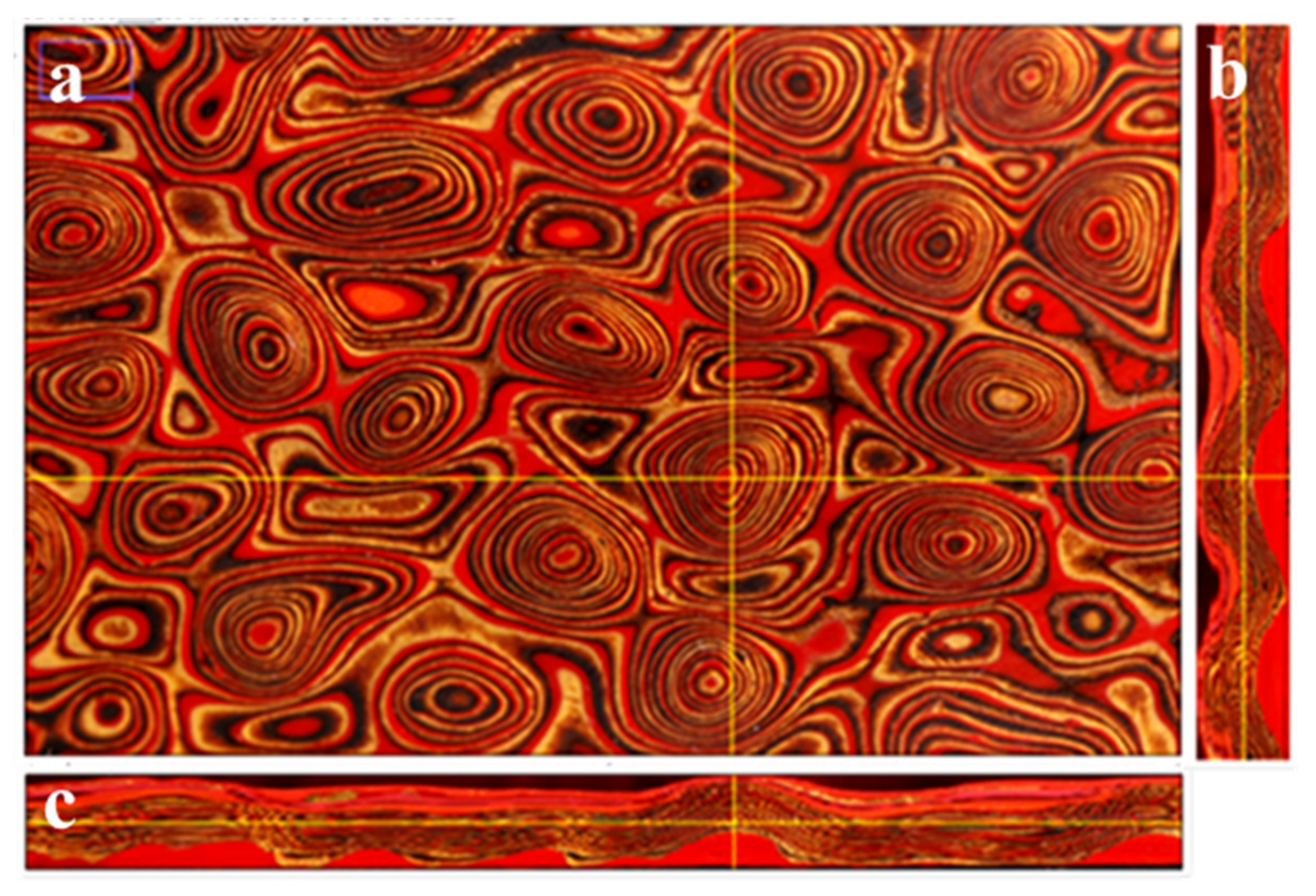The image is an intricate abstract artwork segmented into three labeled sections: A, B, and C. The primary section, A, positioned at the top left, is a dominant rectangle featuring a psychedelic pattern of concentric circles in vivid red, yellow, tan, and black hues. It evokes a 70s vibe with its wave-like motion and layered, almost wood knot-like texture. This section is bisected by a prominent yellow line running vertically and horizontally, giving it a structured yet chaotic feel.

Section B is a narrow, vertically-oriented sliver on the right side of the image. It prominently displays a red and black wave pattern, devoid of circles, mimicking the look of sea waves. A yellow vertical line splits this section as well, connecting it visually with sections A and C.

Section C runs horizontally along the bottom of section A, forming a wide but short rectangle. It features a similar wave pattern to section B, with tight layers of red, yellow, and black that resemble calm ocean waves or geological cross-sections. It too is bisected by a yellow line, continuing the motif from sections A and B.

All three sections are interconnected through these yellow lines, which seem to serve a structural or scale-related purpose, enhancing the layered, psychedelic, and abstract nature of the artwork.